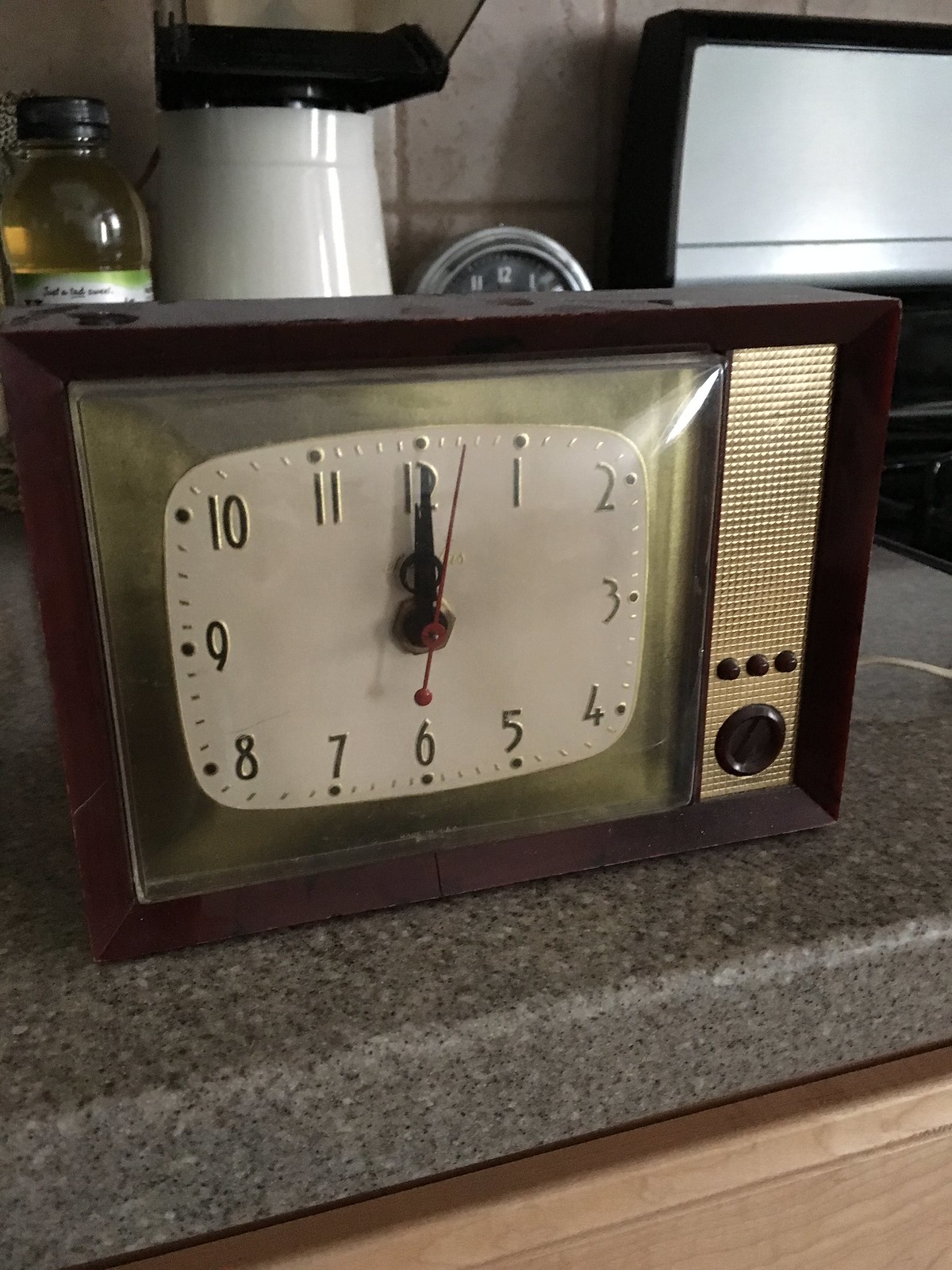A stunningly detailed vintage-style clock that evokes the aesthetic of an old-fashioned television set. The clock's exterior is crafted in a rich brown color with elegant gold accents, adding to its nostalgic charm. Shaped like an antique TV, it features knobs and buttons reminiscent of those classic devices, enhancing its retro appeal. The clock face itself is a rounded rectangle set against a shiny gold metallic background, with raised lines, dots, and numbers also in metallic gold, suggesting a sense of embossment. The hands of the clock are plain black, while the second hand stands out in a vibrant red. This piece sits on a kitchen counter, subtly illuminated by natural light streaming in from a window on the right, highlighting its intricate details and timeless design.